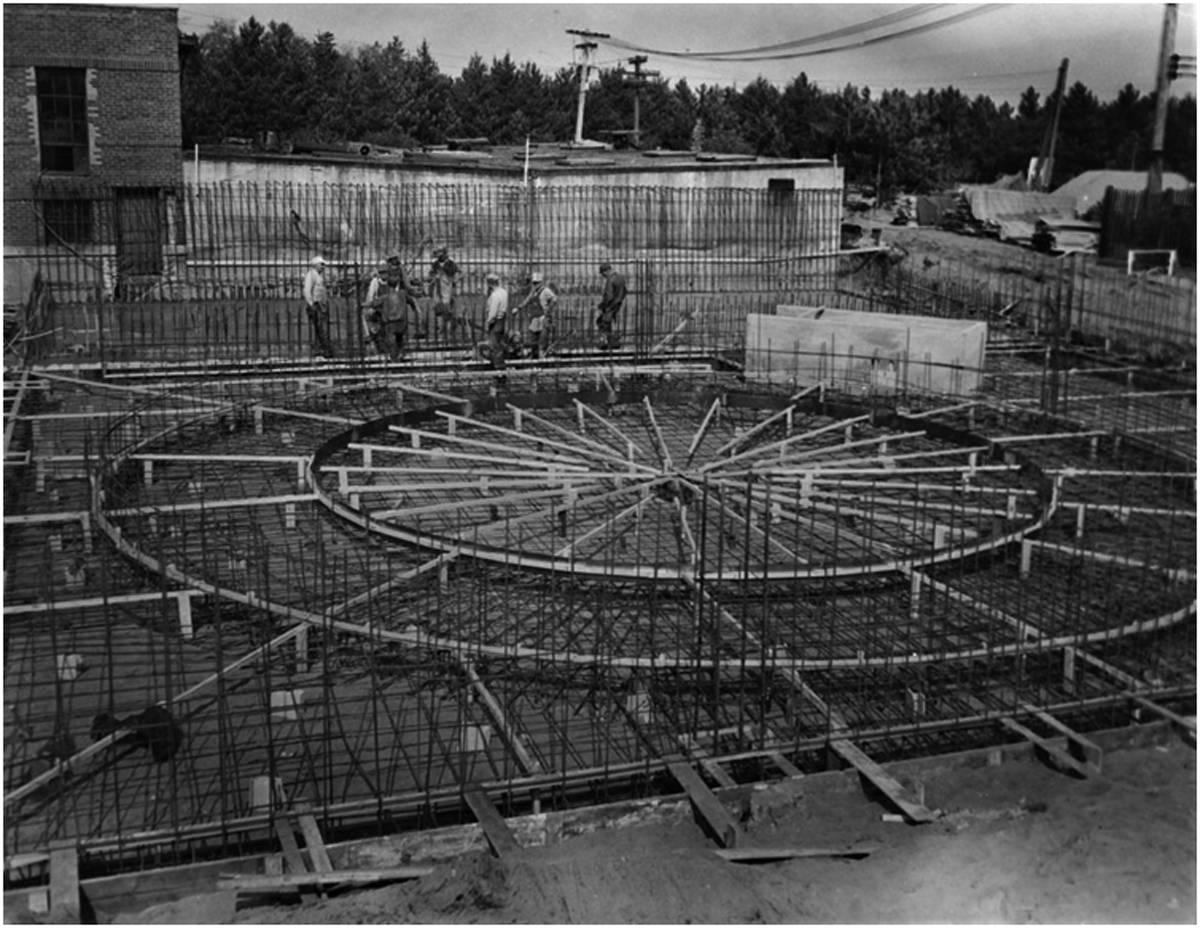This black-and-white, slightly grainy photograph features a construction site dominated by a large, circular framework resembling a wagon wheel or Ferris wheel. The structure has multiple concentric circles and is composed of white-looking beams interspersed with metal rods, likely rebar, suggesting preparation for concrete pouring. The rebar and beams create a striking radial pattern from the center outward. Surrounding this central structure are numerous workmen, approximately ten, busy with different tasks. The background includes a mix of elements: a white rundown building on the upper left, a brick two-story building, a series of power lines and telephone poles, and a landscape dotted with large evergreen trees. The sky above is a whitish gray, completing the monochromatic scene.